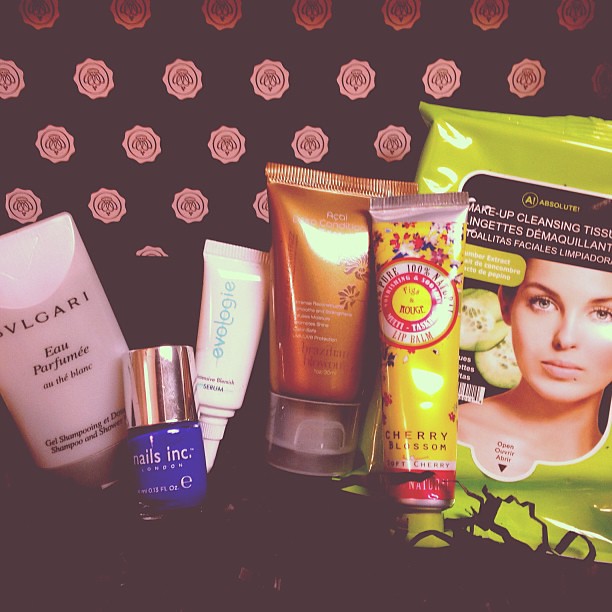This color photograph depicts a meticulously arranged small group of skincare and beauty products, presented in a setting reminiscent of an advertisement. The background consists of a brown fabric adorned with small pink roses. From left to right, the display includes a pink, wide, short tube labeled Bulgari Eau Parfumée au Thé Blanc lotion gel. Adjacent to it is a small round glass bottle of blue nail polish with a golden cap, marked Nails Inc. Next in line is a very small white squeeze tube labeled Evology. Following that is a bronze-colored tube embellished with flowers, the contents of which are indistinguishable. To its right is a yellow squeeze tube with cherry blossom motifs, identified as Cherry Blossom Lip Balm. Finally, on the far right, there is a large square plastic package of makeup cleansing tissues, featuring an image of a woman's face and cucumber slices. The backdrop at the top of the image appears black with white, intricate, seal-like symbols, complementing the aesthetic of this beauty product ensemble.